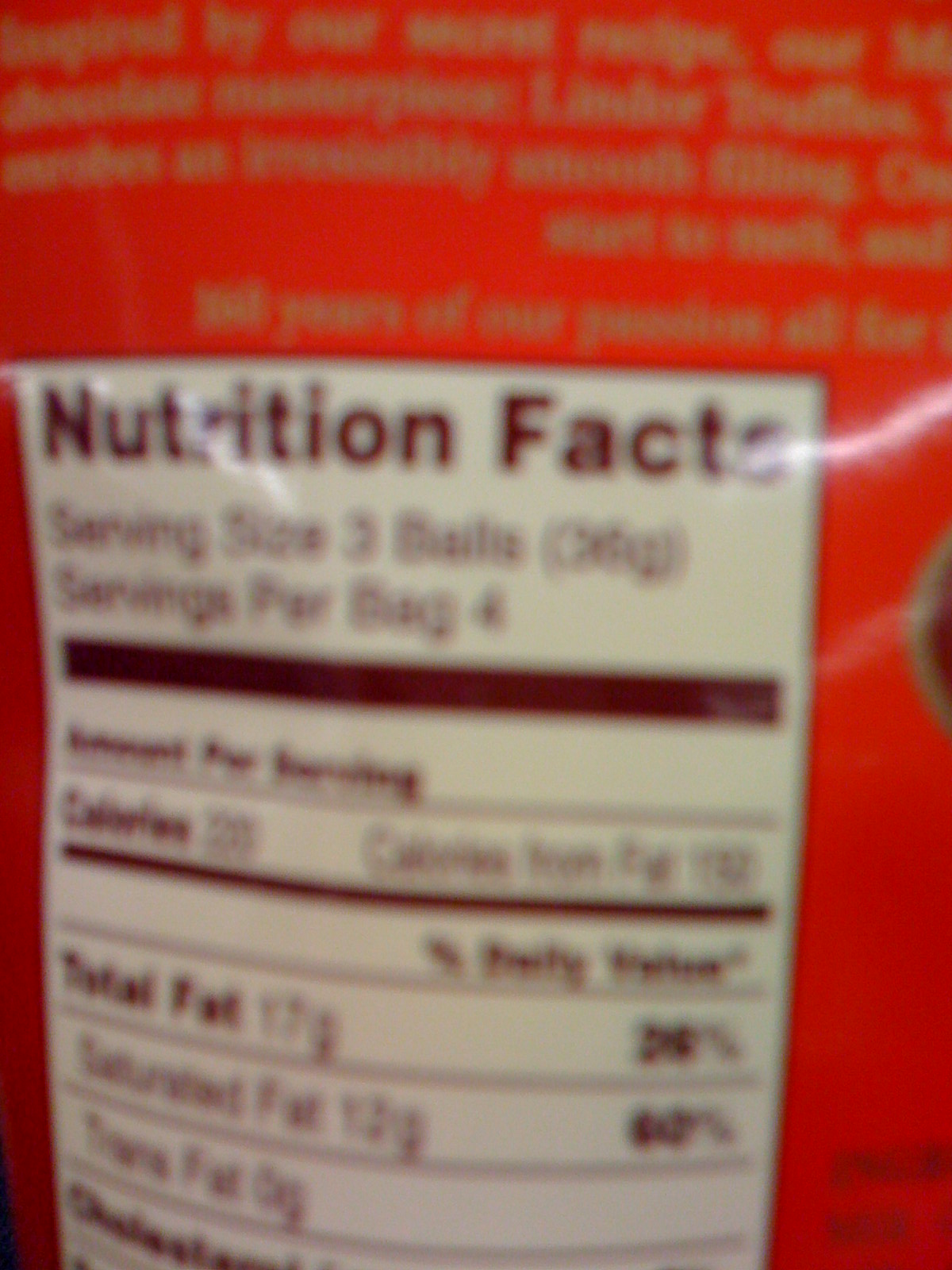This image is a blurred, close-up of a Nutrition Facts label on a red and gold-colored package, likely for a type of truffle or chocolate product. The label has a white background with black text and a black border. The information on the label is somewhat difficult to read due to the blurriness, but it clearly lists details such as serving size, which is 3 balls, and nutritional content including 220 calories, total fat of 17 grams, saturated fat of 13 grams, and 0 grams of trans fat. The top of the label shows the serving size and servings per bag (436 grams). The package design features some maroon and brown elements on the right side, indicating a curve or edge of the design. Reflections of light are visible around the text "Nutrition Facts," making some parts harder to read. The text at the bottom right of the image is too blurred to discern.